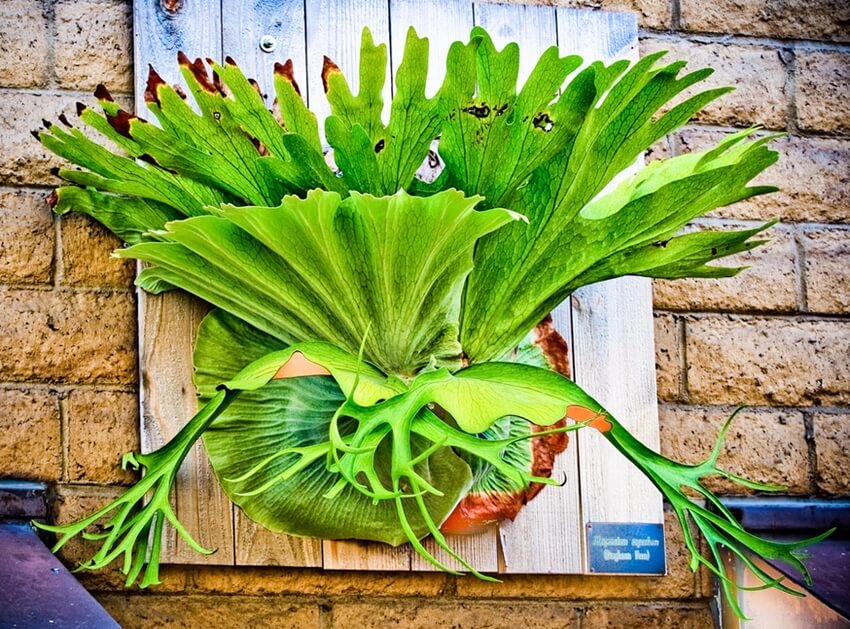This image depicts a vibrant green plant, resembling an air plant or leafy vegetable like lettuce, hanging from unfinished light pine wooden planks, which are affixed to a mud-colored, light orange stone brick wall. The plant's textured and lined leaves flare out in various directions, with brown spots along the edges and some small branches poking out at the bottom. A label with indiscernible white writing on a blue background is attached at the lower right corner of the planks. The plant appears unusually well-preserved, possibly through some form of preservation technique. Metal bars are visible at the lower left and right corners of the planks. Additionally, there's a black countertop-like structure on both sides of the plant. The image, potentially AI-generated due to anomalies among the lower leaves, exudes a surreal quality as plants do not typically grow in such a manner from walls and planks.